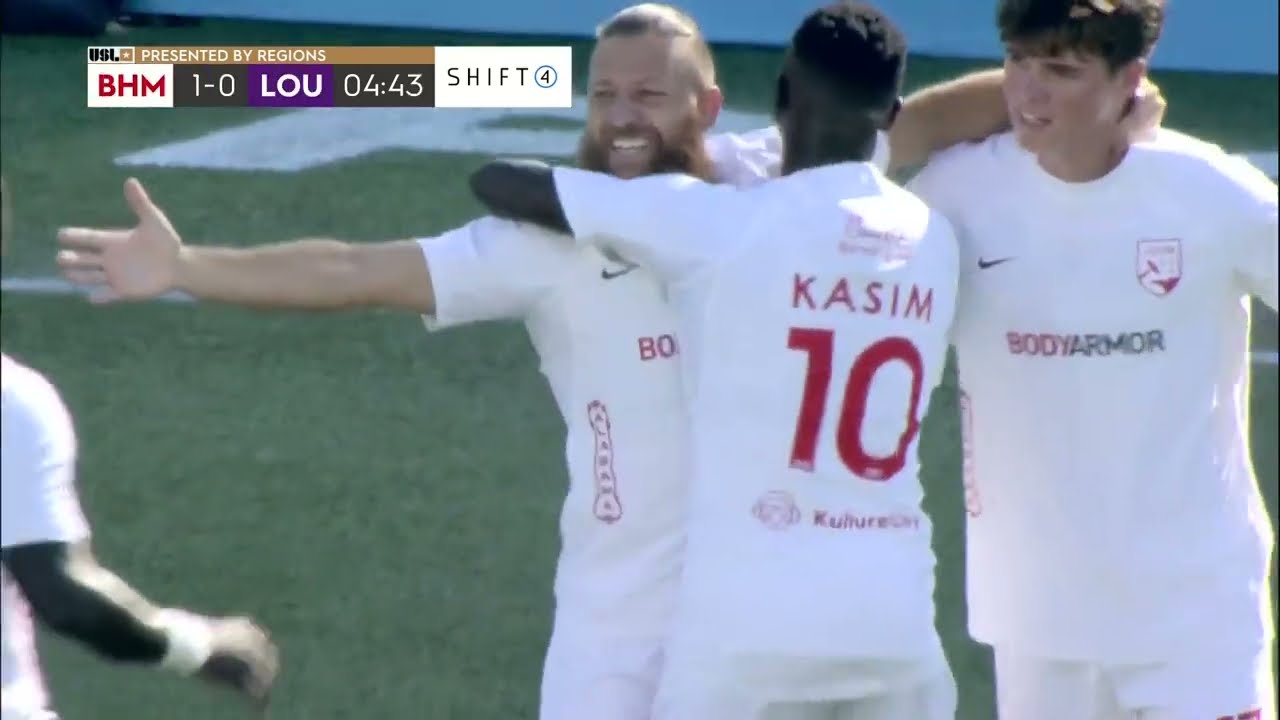The image appears to be a lower-quality screenshot taken from a TV broadcast of a soccer game. It features three men wearing white jerseys with the words "Body Armor" and a Nike checkmark on the left side. In the center, one player, a black man with the name "Kasim" and the number "10" on his back, is hugging another player. The man on the right, who has brown hair, is gesturing to someone off-screen while smiling, inviting them to join the group hug. An additional arm extends from the lower left of the image, partially cut off. In the upper left corner, there is a long black box with various labels and text: "USL" in black font, a thin tan line with "Presented by Regions," followed by "BHM" in red, "1 to 0" in black, "LOU" in purple, a timer reading "04:43" in black, and finally "Shift 4" in white.